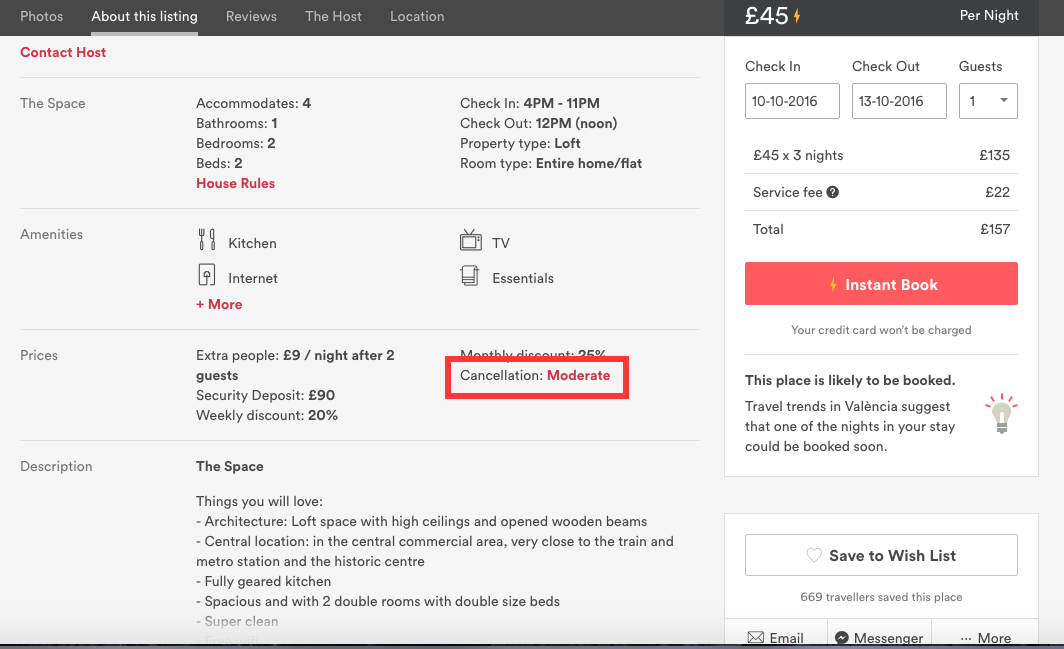Screenshot of a Web Page:

At the top of the webpage, there is a thin black bar extending across the entire width of the screen. Below this bar, the page is sectioned into various categories. Here are the details:

1. **Photo Category**: The first category listed.
2. **About This Listing**: The second category, highlighted with a bar underneath and dark white letters.
3. **Reviews**: The third category.
4. **The Host**: The fourth category.
5. **Location**: The fifth category.
6. **Pricing Symbol**: A British Pound symbol (£) followed by "45" and a small flash symbol, with "per night" to its right.

Towards the top right of the page, there is an option to **Contact Host**.

The main content area consists of four sections:
1. **The Space**: Describes the accommodation details:
   - Sleeps 4 people
   - 1 Bathroom
   - 2 Bedrooms
   - 2 Beds
   - House Rules: Highlighted in red, clickable
   - Check-in: 4 PM to 11 PM
   - Check-out: 12 PM Noon
   - Property Type: Loft
   - Room Type: Entire Home/Flat

2. **Amenities**: Listed with corresponding icons:
   - **Kitchen**: Represented by a fork and knife icon
   - **Internet**: Represented by a plug icon
   - **More Amenities**: Indicated with a "plus more" label in red
   - **TV**: Represented by a TV icon
   - **Essentials**: Represented by a towel bar and towel icon

3. **Prices**:
   - Extra People: £9 per night after two guests
   - Security Deposit: £90
   - Weekly Discount: 20%
   - Monthly Discount: 25%
   - Cancellation: Moderate (Highlighted with a red bar)

4. **Description**:
   - Title: "Things You Will Love"
   - Bullet Points:
     - Architecture: Loft space with high ceilings and open wooden beams
     - Central Location: In the central commercial area, very close to the train and metro station in the historic center
     - Additional bullet points not fully visible

On the right side of the page, there is a vertical rectangular box for booking, including:
   - Check-in: 10 October 2016 (10-10-2016)
   - Check-out: 13 October 2016 (13-10-2016)
   - Guests: Highlighted as 1 guest
   - Cost Breakdown:
     - £45 per night for 3 nights: £135 total
     - Service Fee: £22
     - Total Cost: £157
   - Booking Button: Red bar labeled "Book"
   - Additional Information: Indicates that the place is likely to be booked, etc.